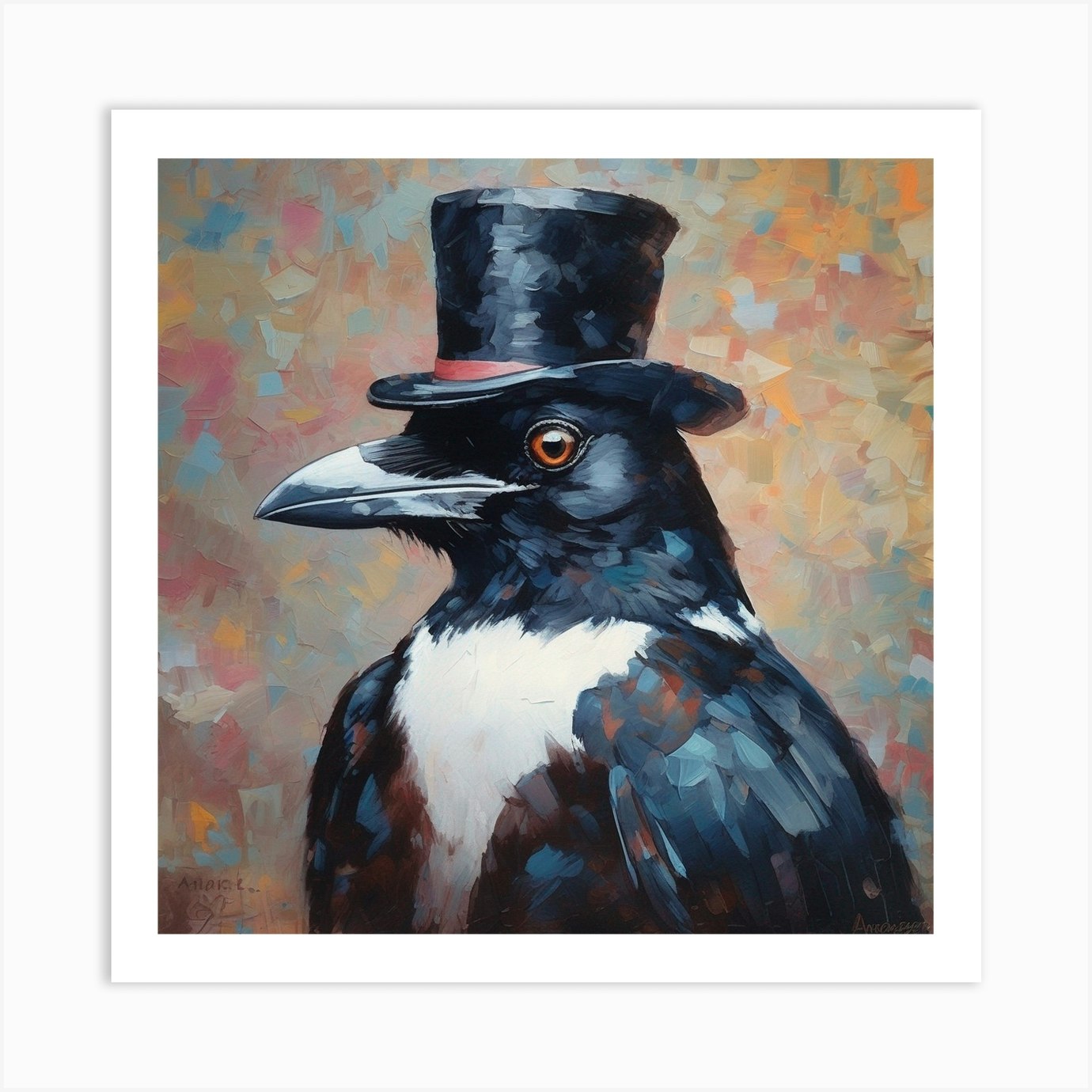This painting depicts a crow adorned in a black top hat with a red ribbon around the rim, showcasing a captivating blend of realism and whimsy. The crow, with its long black beak and rust-colored, open eye, sits against a backdrop filled with an explosion of color through thick, expressive brush strokes. The bird's dark feathers — exhibiting shades of black, dark blue, and some brown — highlight the artist's ability to capture the iridescent qualities inherent in an actual crow's plumage. Below its neck, the crow displays a distinctive white, triangular breast, adding a striking contrast. The crow appears almost posed, as if sitting for a portrait, emphasizing its dignified yet comical aura. The background consists of smudged tones of light beige, orange, pink, light blue, cream, yellow, and mauve, set within a white frame that captures the crow from the chest up. The painting makes use of heavy, thick brush strokes to create a textured, almost tangible quality to the feathers and surroundings, enhancing the overall vivid and dynamic nature of the artwork.